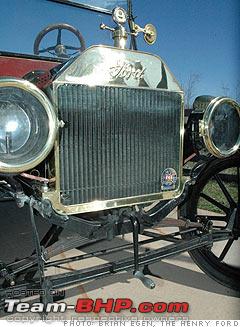The image captures a close-up view of the front section of a vintage red Ford vehicle, likely from the 1920s. Prominently displayed in the center at the bottom of the silver square grille is a classic crank handle used for starting the car. On either side of the grille, there are large, old-fashioned headlights, and traditional tires can be seen peeking from the sides. Above the grille, the word "Ford" is laminated, and a clear blue sky is visible through the car's window and above the steering wheel, indicating a sunny day. The text on the image indicates its source, stating "Photo Brian Egan, The Henry Ford" along with a watermark reading "teambhp.com" – with 'team' in white letters and 'bhp.com' in red letters – suggesting it is a copyrighted image.